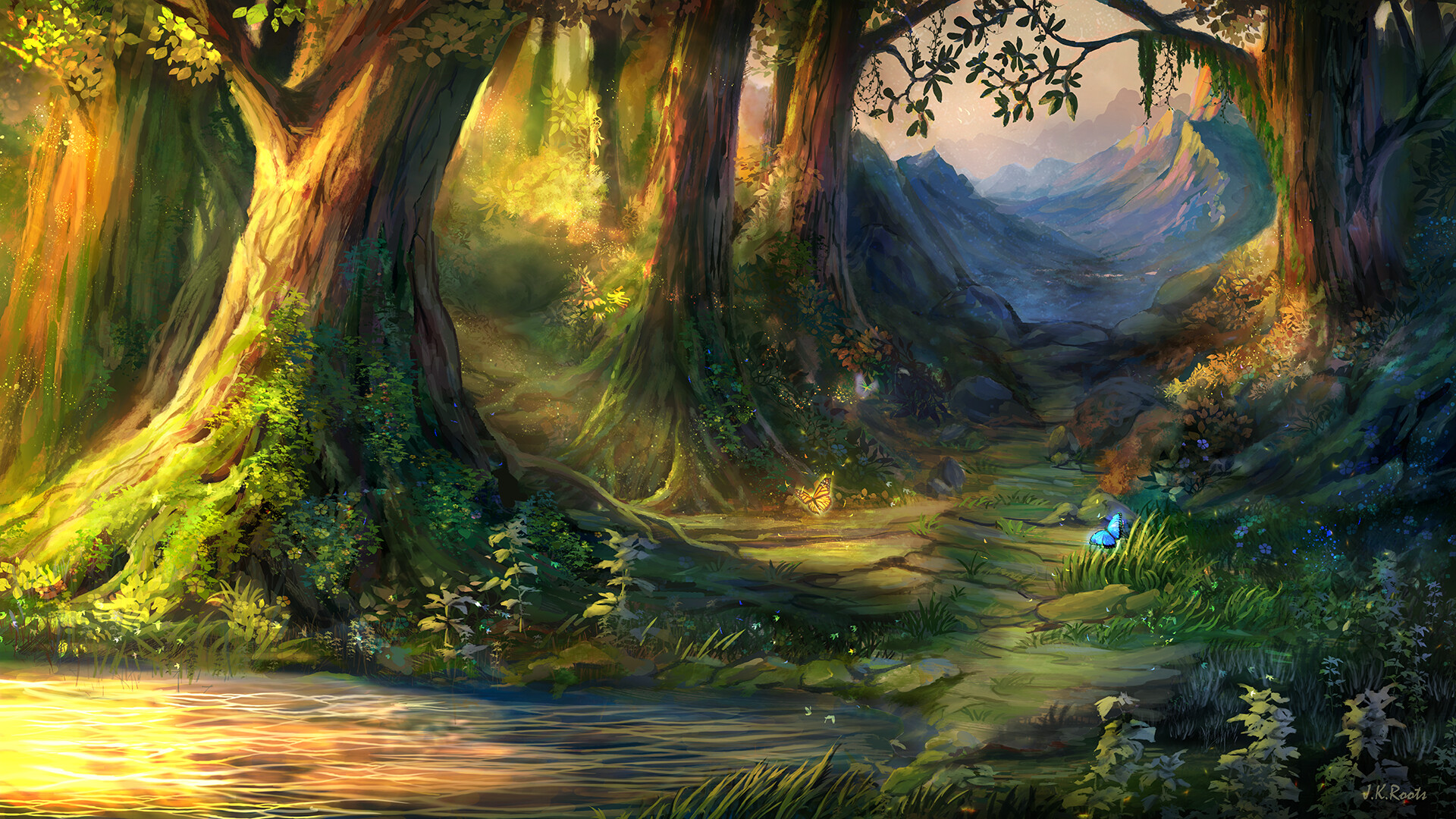This vibrant and detailed illustration depicts a magical, mythical forest bathed in golden sunlight streaming from the left. The foreground features tall, thick trees draped in moss and adorned with various plants and flowers, creating a lush, verdant scene. A shimmering pool of water on the bottom left catches the sun's reflection, enhancing the serene beauty of the setting. A path, covered in green and yellow hues, winds through the forest, guiding the viewer's eye towards the background where rocky, mist-covered mountains, appearing in shades of blue and purple, rise against a darker, clouded sky. Blue butterflies flit about, with one perched on the grass to the right, adding a touch of whimsy to the scene. The composition is dominated by the towering trees and dense foliage, which frame the ethereal landscape beyond. The artwork is signed "JK Roots" in the bottom right-hand corner, suggesting the artist's signature.